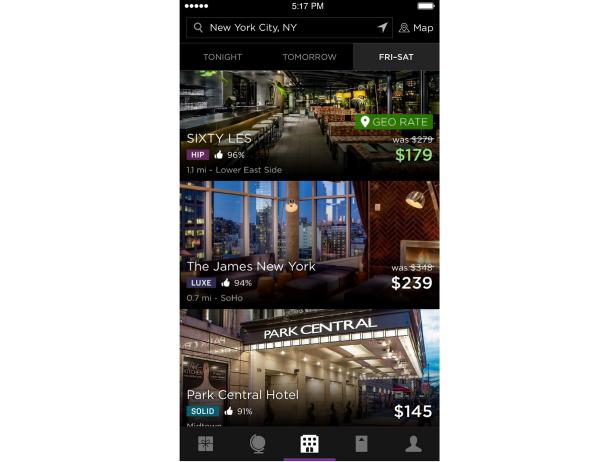The image depicts a smartphone screen displaying a room rental app with details about available accommodations in New York City. 

The phone shows the current time as 5:17 p.m. and has full signal bars and battery life. The screen features a sleek black background. At the top, it indicates the location as "New York City, New York," and there is an interactive map for navigation.

Below, there are three listings for accommodations:

1. **60 LES** 
   - Price: Was $279, now $179 (Geo rate)
   - Rating: 96% with a thumbs-up icon
   - Distance: 1.1 miles from Lower East Side
   - Availability: Tonight, Tomorrow, Friday, Saturday

2. **The James, New York**
   - Price: Was $349, now $239 (Lux rate)
   - Rating: 94% with a thumbs-up icon
   - Distance: 0.7 miles from Soho
   - Availability: Tonight, Tomorrow, Friday, Saturday
   
3. **Park Central Hotel**
   - Price: $145 (Solid rate)
   - Rating: 91% with a thumbs-up icon
   - Distance: Not specified
   - Availability: Tonight, Tomorrow, Friday, Saturday

Each listing includes a photo of the property with relevant details overlaid in white and blue fonts.

At the bottom of the screen, there is a navigation bar with various icons, potentially representing features such as a gift box with a bow, a globe, a grid of six squares, a calculator-like icon, and a person.